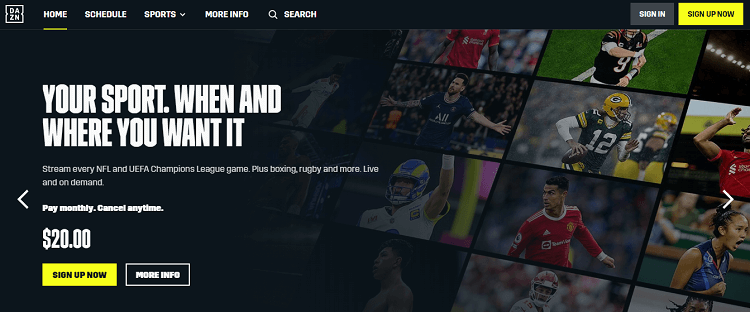The image displays a user interface of a sports streaming platform, with a navigation bar at the top. On the top left, there is a logo reading "DAZN" inside a box. The navigation bar includes several menu items: "Home," "Schedule," "Sports" (which features a drop-down button), and "More Info." A search bar with a magnifying glass icon is also present. The "Home" menu item is highlighted with a yellow underline.

Additionally, there are two buttons on the right side of the navigation bar: a gray "Sign In" button and a yellow "Sign Up Now" button.

Below the navigation bar, prominently displayed in large white capital letters is the slogan: "YOUR SPORT, WHENEVER YOU WANT IT." The platform promises access to live and on-demand streaming of every NFL and UEFA Championship League game, plus boxing, rugby, and more. 

Beneath this message, pricing information indicates that users can "Pay monthly, cancel anytime" for $20. The call-to-action is reinforced with another yellow "Sign Up Now" button and a black "More Info" button below.

The lower part of the interface features images of various athletes, including football players, soccer players, and track stars, emphasizing the diverse sports content available on the platform.